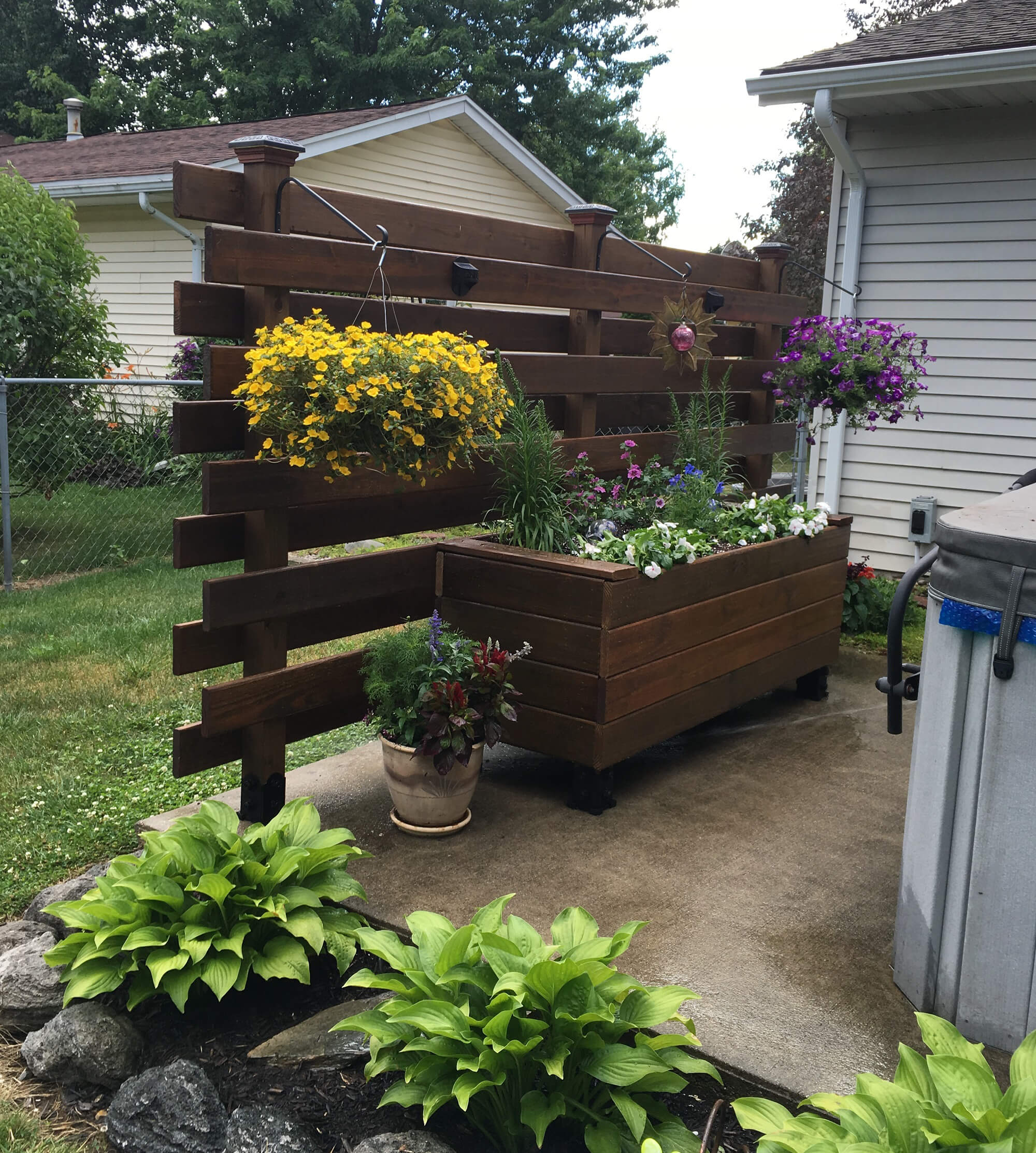The photograph captures a well-tended backyard garden area dominated by various flowering plants. The centerpiece of the scene is a wooden planter containing a vibrant mix of blue, white, and purple flowers, positioned prominently on a concrete slab. Behind this planter stands a wooden backdrop adorned with hanging plants featuring yellow and purple blooms, alongside a star-shaped decorative object with a shimmering purple reflective ball at its center. Adjacent to the wooden planter is a plastic pot housing a fern and a plant with striking reddish-brown leaves.

In the background, the exterior of a house with gray vinyl siding is visible, hinting at a residential setting. The edge of a roof can be seen, suggesting a bungalow-style home. To the left, there's a chain-link fence bordering the property, separating it from another building clad in beige vinyl siding. A couple of trees enhance the greenery of the scene. In the foreground, green plants are rooted in the lawn, adding to the lushness of the garden. A small corner of what appears to be a hot tub peeks into the frame, further enriching the cozy and inviting atmosphere of this backyard oasis.